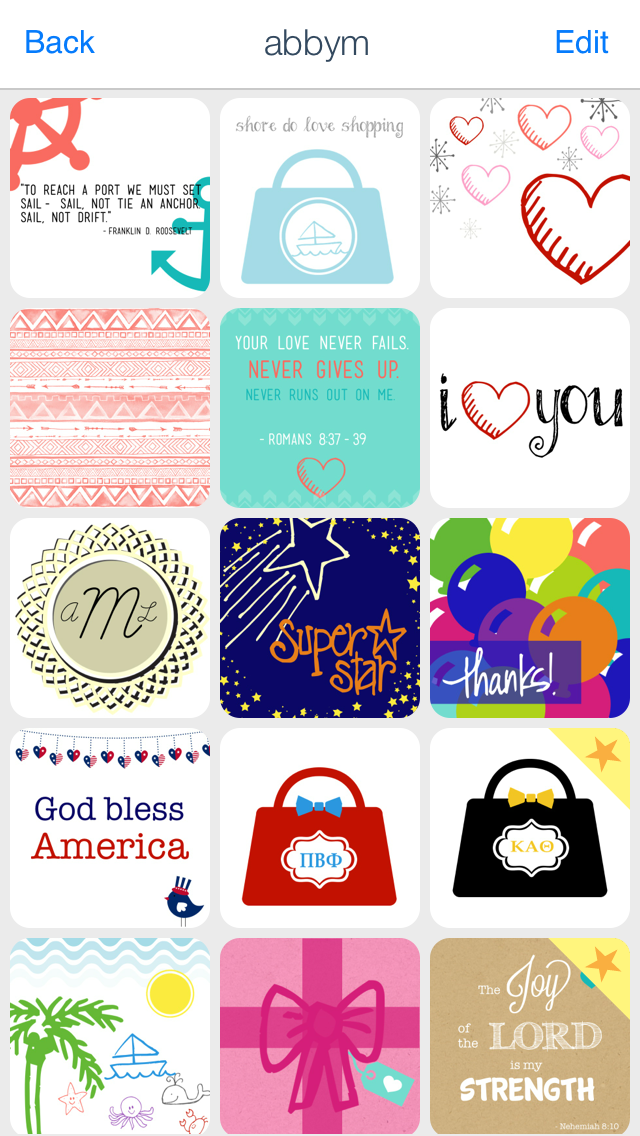The image is a screenshot of a mobile app interface showcasing a digital collection of cards or images organized in a grid layout. At the top, there is a back button, followed by the user name "Abby M" centered, and an edit button on the top right. Below this header, there is a grid layout consisting of 15 digital cards arranged in five rows and three columns.

- **First Row:**
  - **Card 1:** Features a nautical theme with a red ship and an inspirational quote: "To reach port, we must set sail. Sail, not tie and anchor; sail, not drift." — Franklin D. Roosevelt.
  - **Card 2:** Displays a light blue handbag icon with a sailboat inside, accompanied by the text, "Sure do love shopping."
  - **Card 3:** Showcases a design with hearts of various sizes and shapes.

- **Second Row:**
  - **Card 1:** Displays a pattern with pink, red, and white geometric shapes and lines.
  - **Card 2:** Features a teal background with an inscription from Romans 8:37-39: "Your love never fails, never gives up, never runs out on me."
  - **Card 3:** A white background with the text "I ♥ you" in black and red, where the heart is creatively drawn.

- **Third Row:**
  - **Card 1:** Exhibits a monogram design with the initials "AML" inside a gold, doily-like circle.
  - **Card 2:** Dark blue background with a yellow star and the text "Superstar."
  - **Card 3:** Card with colorful balloons and the text "Thanks" in the foreground.

- **Fourth Row:**
  - **Card 1:** White background featuring a string of hearts and American flags, along with the text "God bless America" and a small bird at the bottom.
  - **Card 2:** Red handbag with a blue bow and a white label with the text "NBO."
  - **Card 3:** Black handbag with a yellow bow and a white label with the text "COW."

- **Fifth Row:**
  - **Card 1:** Illustrative scene with palm trees, the sun, a whale, and a boat, invoking a tropical beach theme.
  - **Card 2:** Pink background with a large pink bow, small hearts, and an envelope icon.
  - **Card 3:** The text "The joy of the Lord is my strength" from Nehemiah 8:10, with a star in the right corner.

Each card in this collection carries unique themes and messages, ranging from inspirational quotes and religious verses to creative designs and patterns.